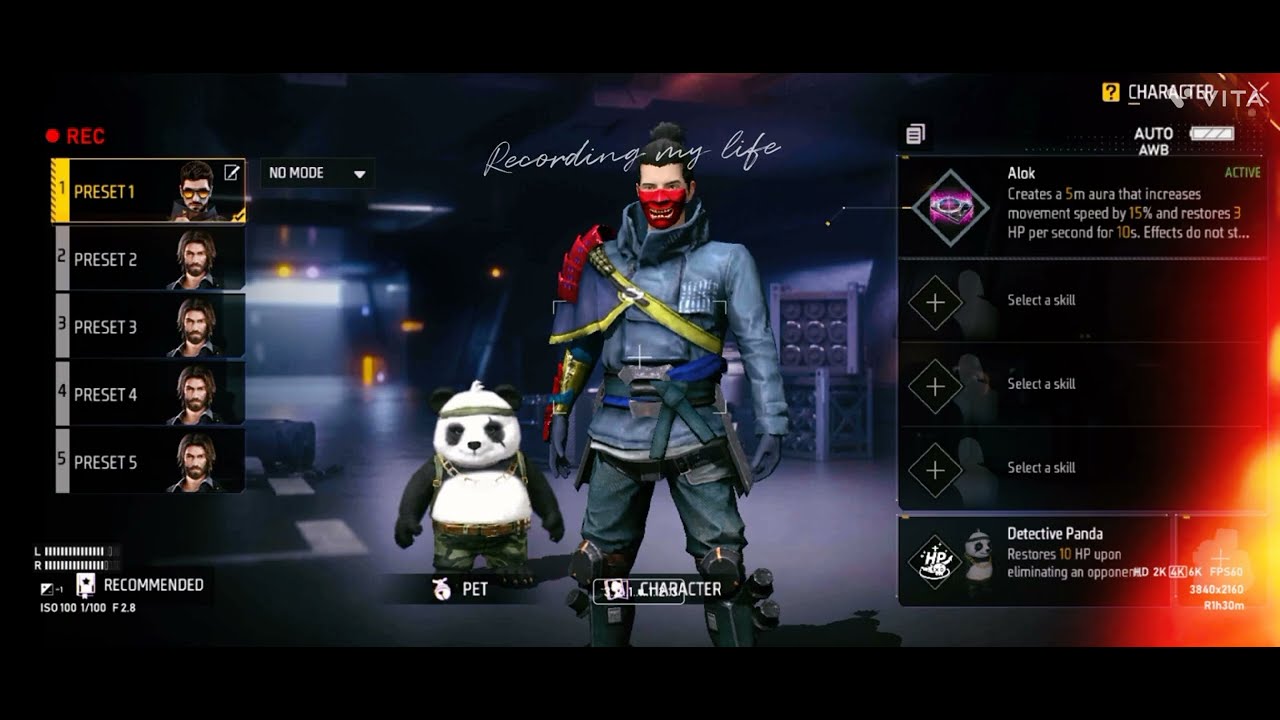The image appears to be a screenshot from a video game displayed on a monitor. The background is predominantly black with dark hues like blues and purples. In the center of the screen stands a male character with a man bun or ponytail, wearing what looks like a blue cargo outfit equipped with various belts and garb, including knee pads, long gloves, and possibly a container for a weapon on his left side. His face is covered with a red handkerchief or mask. The text "recording my life" is superimposed over him. To his right stands a small panda bear labeled as "pet." 

On the left side of the screen, there are five character images labeled "preset" from 1 to 5, with preset 1 highlighted in yellow font while the others are in grey. Each preset depicts characters that are mostly identical, except for the first one. Additionally, the game is annotated as recommended ("R for recommended") at the bottom of this list. On the right side, notable text includes "select a skill," "detective panda," and other similar menu options, possibly part of an interface for modifying the character. The edges of the screen feature black horizontal bars at the top and bottom, and what appears to be a chat room panel on the right side.